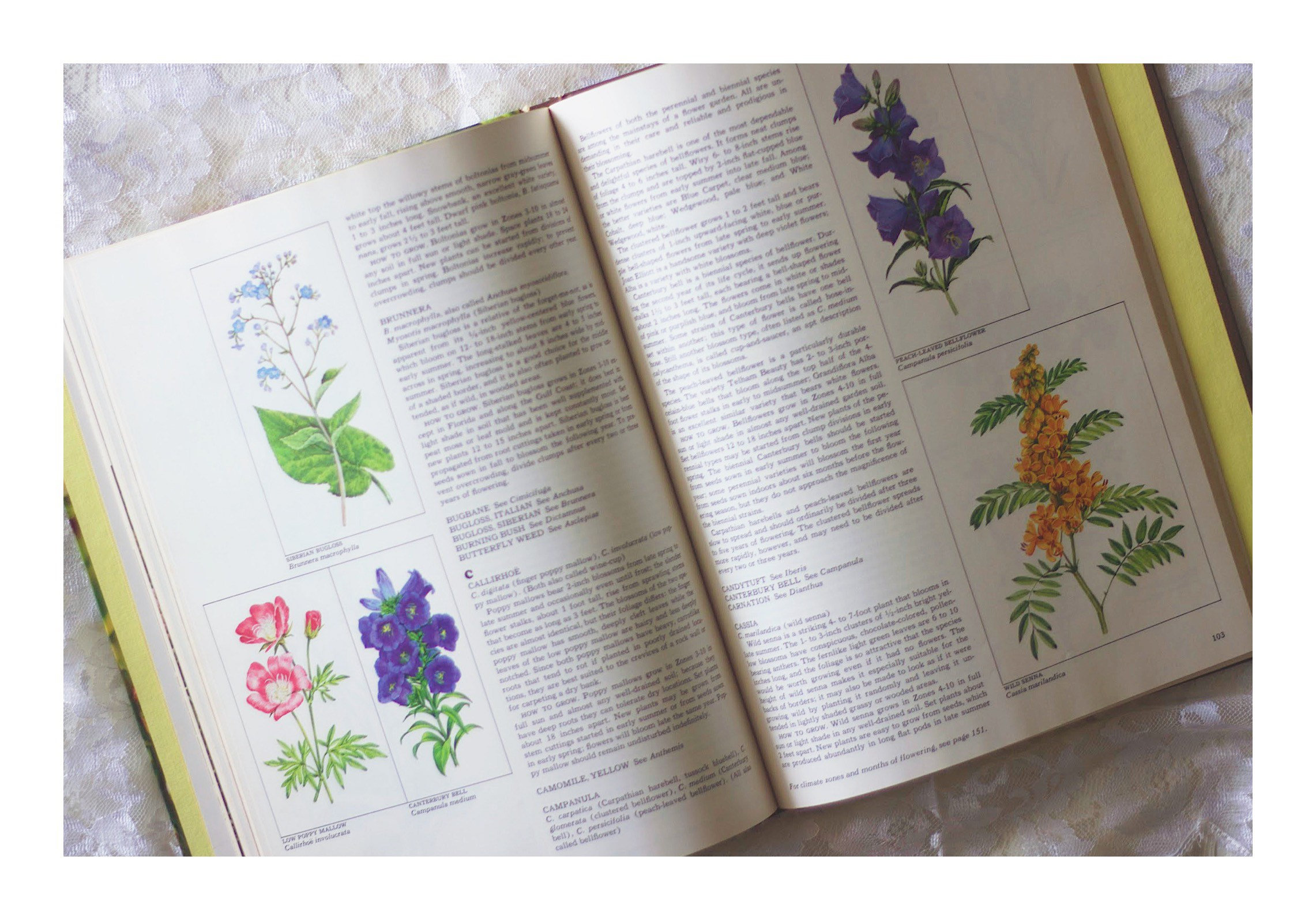The image depicts an open book on a bright, naturally lit, and textured white surface. The book, which is in full color and very clear, features various types of flowers across two pages. The left page shows three images of flowers in the left column, specifically some pink, purple, and blue blossoms, accompanied by descriptive paragraphs in the right column. The right page, which is labeled as page 103, reverses this layout with descriptive text in the left column and two images of flowers—purple and orange—in the right column. The book is slightly tilted diagonally counterclockwise, and no other objects are visible in the image.